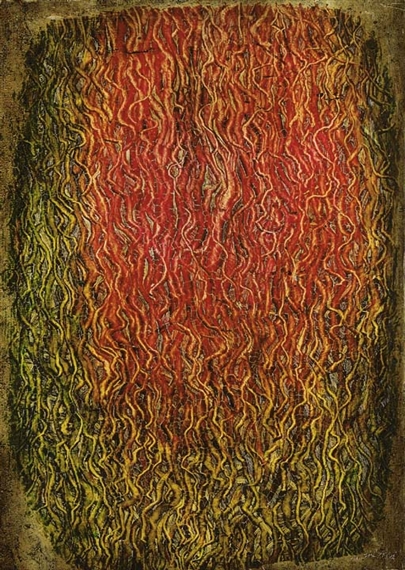The abstract artwork features an intricate composition that evokes a sense of organized chaos. The painting consists of a multitude of string-like or spaghetti-like strands, meticulously arranged to form a roughly rectangular shape. The outer edges of the piece are characterized by dark, almost frayed borders in hues of black, dark grey, and dark green. Moving inward, these strands gradually transition into a spectrum of vibrant colors, with dark green at the periphery giving way to shades of yellow. Towards the top center, the strands become more dynamic and exhibit a fiery mixture of red, yellow, and orange, culminating in a dense core of these warm colors. Amidst this colorful mass, the very center reverts back to a darker palette, blending black and dark grey hues. The edges of the image suggest a fraying effect, adding to the texture and depth of the piece. The entire composition gives an impression of organic, fluid movement, reminiscent of both tangled grass and a plate of spaghetti, making it a unique visual experience.